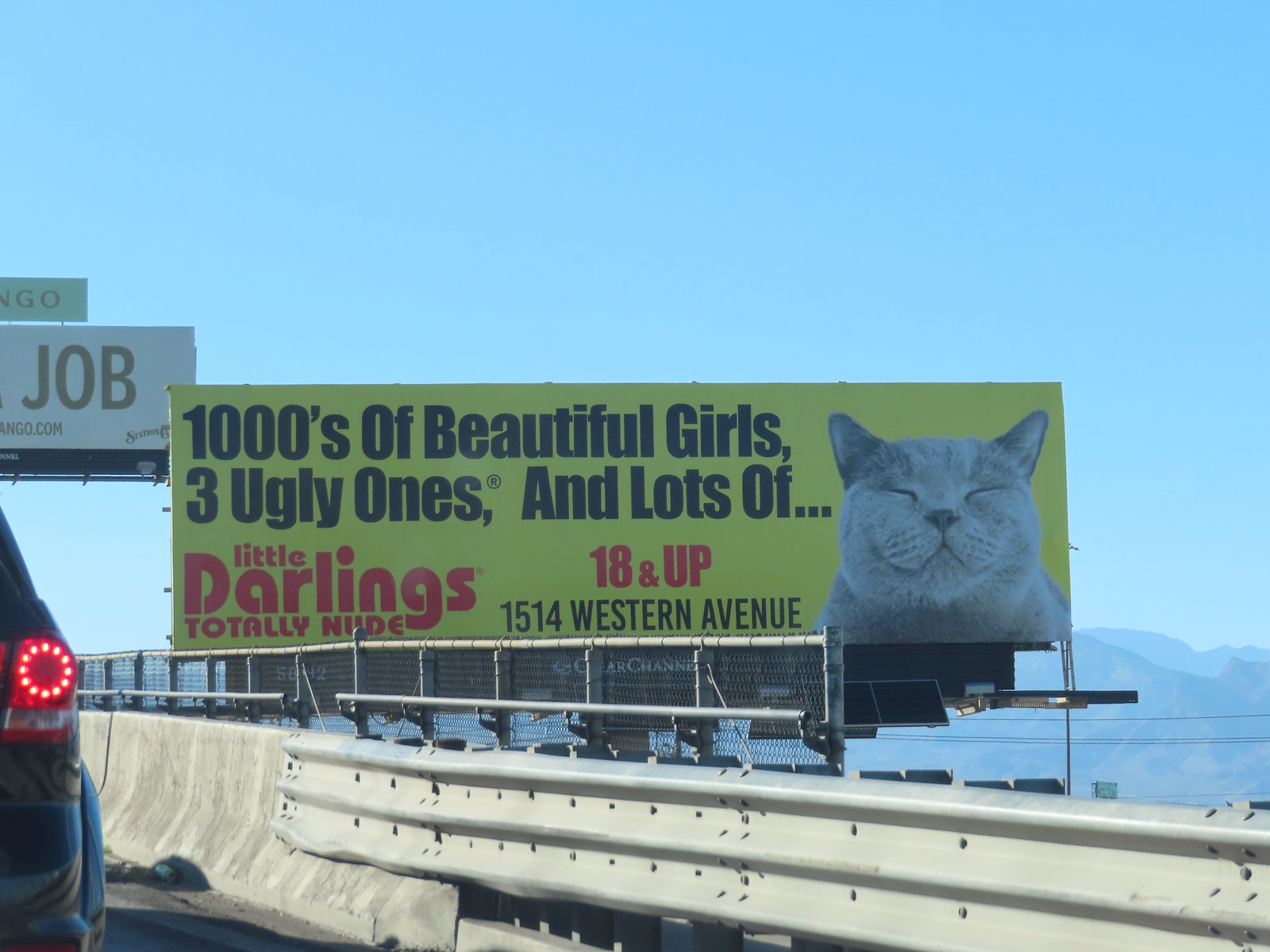This photograph, taken from inside a car through the windshield, captures a broad scene of a roadway that seems to be on a highway overpass or bridge. The bridge, made of concrete with a visible railing, spans a river. On the right, a steel guardrail runs alongside the road. Up above, the sky is a clear, beautiful blue, and in the distance, a mountain range can be seen.

Dominating the scene is a large billboard prominently positioned near the road. The billboard features a striking yellow background with the image of a smiling gray cat on the right side, showing just its face and shoulders. The black text on the billboard reads: "Thousands of beautiful girls, three ugly ones, and lots of..." leading to the cat's image. Below this, in red text, it states, "little" in small print and "darlings" in very large print, followed by "totally nude." Also in red text to the right, it says, "18 and up," and in black text below, "1514 Western Avenue." This suggestively provocative advertisement gives off a strong impression of being from Florida.